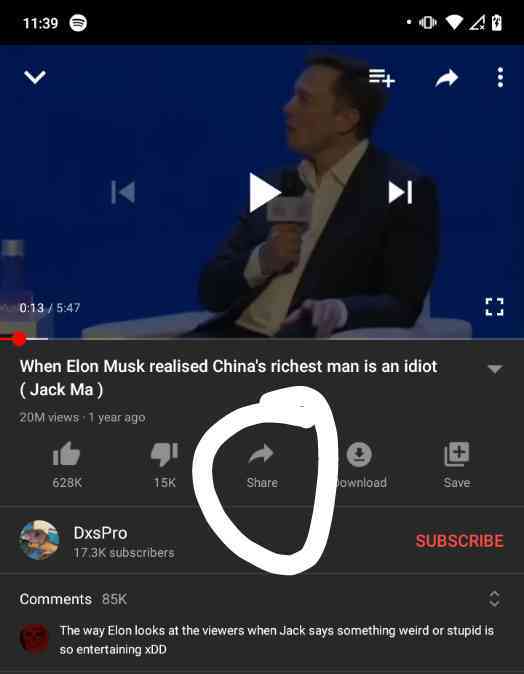This image is a screenshot of a mobile phone displaying a YouTube video. The top of the screen features a black status bar indicating the time as 11:39, along with icons for Wi-Fi connectivity, signal strength, and vibration mode. The battery indicator is also visible.

Centered below this is a still from the video, showing Elon Musk seated on a white chair against a blue background, likely at a conference. He is holding a microphone in his right hand, wearing a blazer and white shirt, and facing towards the left side of the screen.

Overlaying the video image are YouTube's video control options, including play/pause buttons and a progress bar. The progress bar shows that 13 seconds of the video have elapsed out of a total 5 minutes and 47 seconds. The video's title is displayed below: "When Elon Musk Realized China's Richest Man Is an Idiot (Jack Ma)." This video has garnered 20 million views since being uploaded a year ago, with 620,000 likes and 15,000 dislikes.

Further controls include marked buttons for sharing, downloading, and saving the video. The share button is notably circled in a hand-drawn thick white line. The video's creator is identified as "DXS Pro," who has 17.3K subscribers. There is also a prominently displayed subscribe button.

Beneath the video details, a comment by a viewer is partially visible, stating: "The way Elon looks at the viewers when Jack says something weird or stupid is so entertaining, XDD." This video has accumulated 85,000 comments.